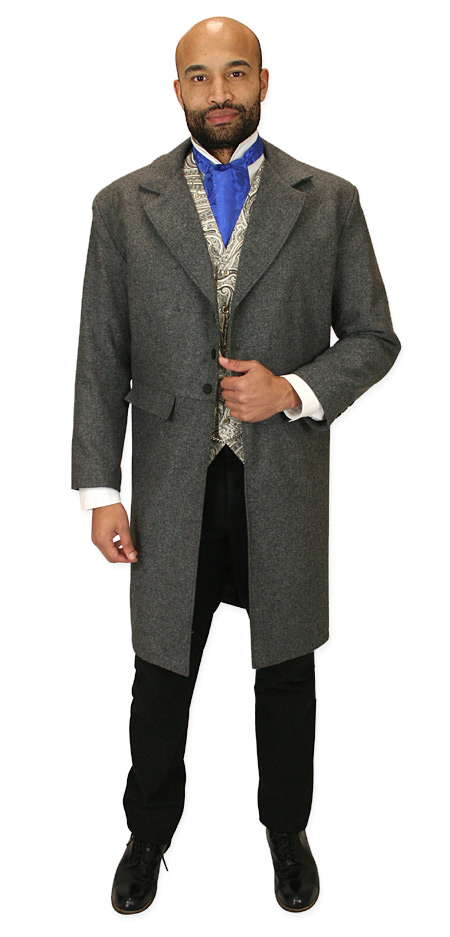The image features an African-American man with a bald head and a thin full beard and mustache. He has dark skin, brown eyes, and brown eyebrows. He is staring straight ahead at the camera with a neutral expression, his lips closed and very slightly smiling. He is dressed in a charcoal gray trench coat-inspired overcoat that reaches just above his knees, with two or three buttons visible. Underneath, he wears a white long-sleeve button-down shirt, the cuffs of which can be seen extending from the sleeves of the coat. Over the shirt, he has on a gold patterned gray vest and a bright blue ascot or tie. His left hand grasps the edge just below the lapel of his jacket, while his right hand rests naturally by his side. He completes his outfit with black dress pants and black laced dress shoes. The background is entirely white, putting all attention on the man's detailed attire and composed demeanor.